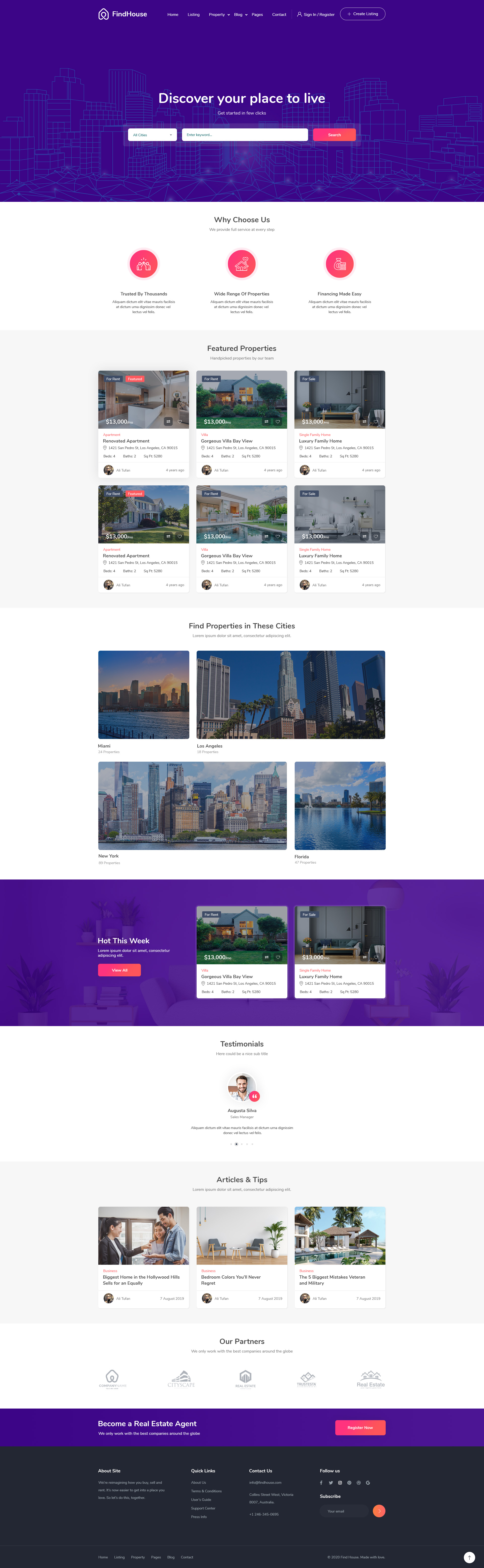**Caption**

This image is a screenshot from a real estate search website, showcasing its user interface. The layout appears to be compressed, making the text slightly difficult to read. Dominating the top section is a purple header bar that contains the site's logo and navigation menu. The menu includes links to 'Home,' 'Listing,' 'Property,' 'Blog,' 'Pages,' 'Contact,' alongside options for users to 'Sign In,' 'Register,' and 'Create Listings.' 

Below the header, the main section features a bold white heading that reads, "Discover Your Places to Live." Underneath, it says, "Get started in a few clicks," accompanied by a dropdown menu labeled "All Cities" for location selection and a search bar prompting users to "Search."

Further down, a section titled "Why Choose Us?" outlines three key benefits of the site: "Trusted by Thousands," "Wide Range of Properties," and "Financing Made Easy." This is followed by a "Featured Properties" area displaying various home listings in a blog-style format, offering both interior and exterior views of the properties.

Towards the bottom, the site highlights a section titled "Find Properties in These Cities," directing users to specific locations. At the very end, there's a segment providing articles and tips related to real estate.